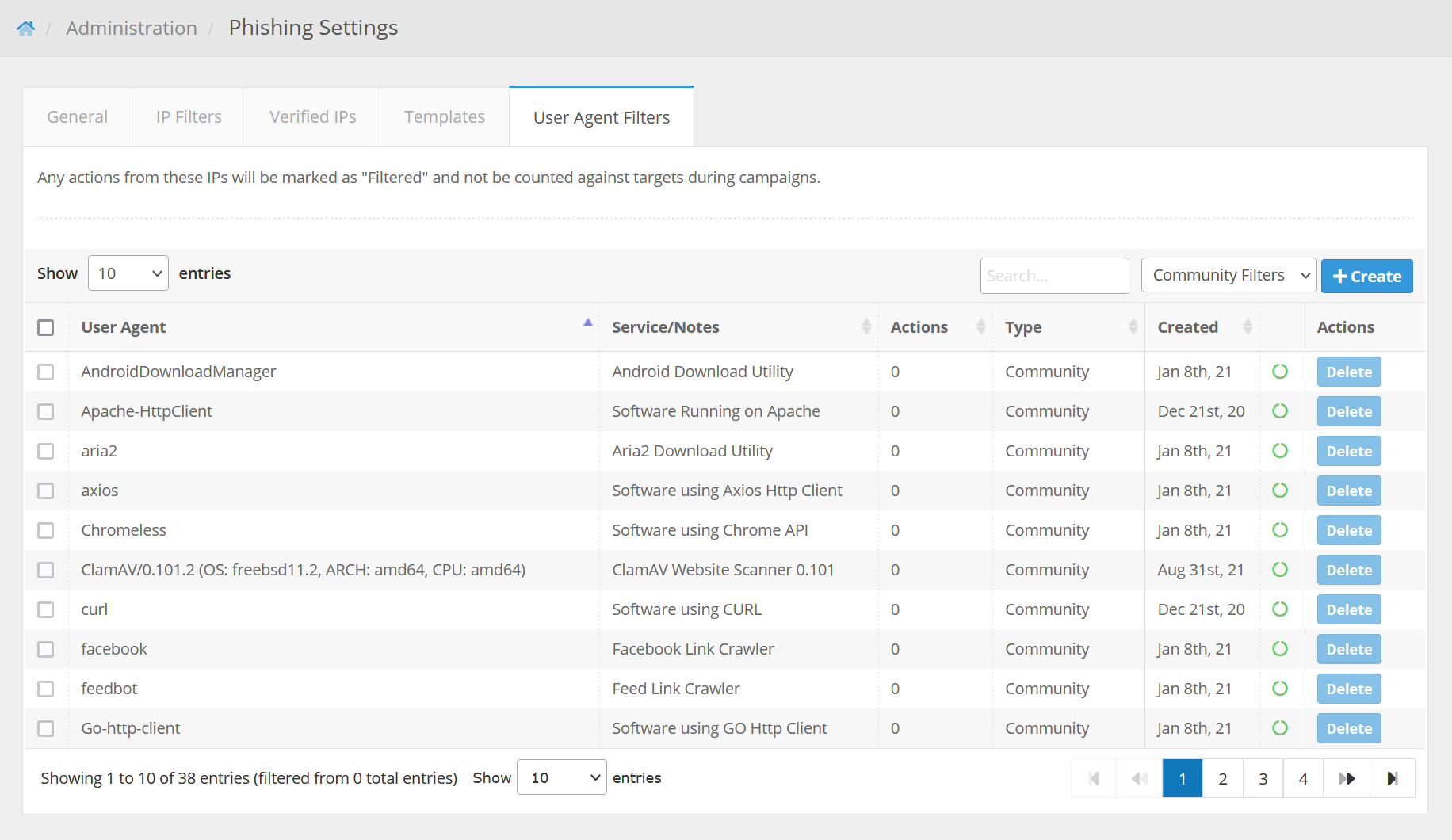Caption: 

The screenshot showcases a webpage with a gray background, displaying various administrative settings related to phishing management and IP filters. At the top, tabs labeled "Administration," "Phishing Settings," "General IP Filters," "Verified IPs," and "Templates" are visible. A distinct blue line highlights the "User Agent Filters" tab. A prominent message states that any actions from the outlined IPs will be "filtered" and not counted against targets during phishing campaigns. 

The interface shows options to "Show 10 entries" and contains a search bar along with a section for "Community Filters." A blue rectangle button labeled "Create" with a plus sign is prominently displayed. Below, the table columns are categorized under "User Agent," "Service," "Notes," "Actions," "Type," "Created," and "Actions," with checkboxes available for each item.

The listed entries include services named "Android Download Manager" and "Apache HTTP Client." The first service is noted as an "Android Download Utility," listed under zero "Community Filters," with a creation date of "January 8th, 2021," indicated by "Jan 8, 21." It features a green circle and an action button labeled "Delete" and "Wipe" in a blue rectangle. Similarly, the "Apache HTTP Client" service entry describes software running on "Apache," also listed with zero "Community Filters," and has a creation date of "December 21st, 2021," shown as "Dec 21, 21." It too has a green circle and a blue action button labeled "Delete" beneath "Actions."